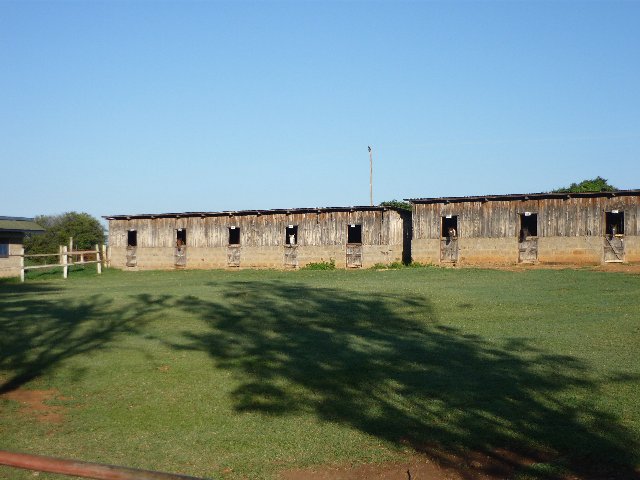The image depicts an old, weathered horse barn divided into two low-rise structures. Each barn features a series of horse stalls with half doors, totaling eight stalls. Five of the stalls have horses poking their heads out, including a distinct brown horse in the second stall on the left building and a white horse in the fourth stall. The barns are constructed from a mixture of gray and brown cinder block at the base, transitioning to weathered gray wood with patches of lighter and darker hues. The roofs are nearly flat with a slight tilt and feature awnings that protect the upper sections from weathering more than the lower parts.

The foreground includes a lush, well-maintained green field resembling a golf course, enclosed partially by a wooden fence. In the background, numerous green trees stand tall against a clear, bright blue sky, indicating a sunny day. Also visible to the left is another outbuilding, more structurally sound and resembling a house, which contrasts with the more makeshift, shack-like appearance of the horse barns. The shadow of a tree casts across the vibrant grass, adding to the scenic rural landscape.